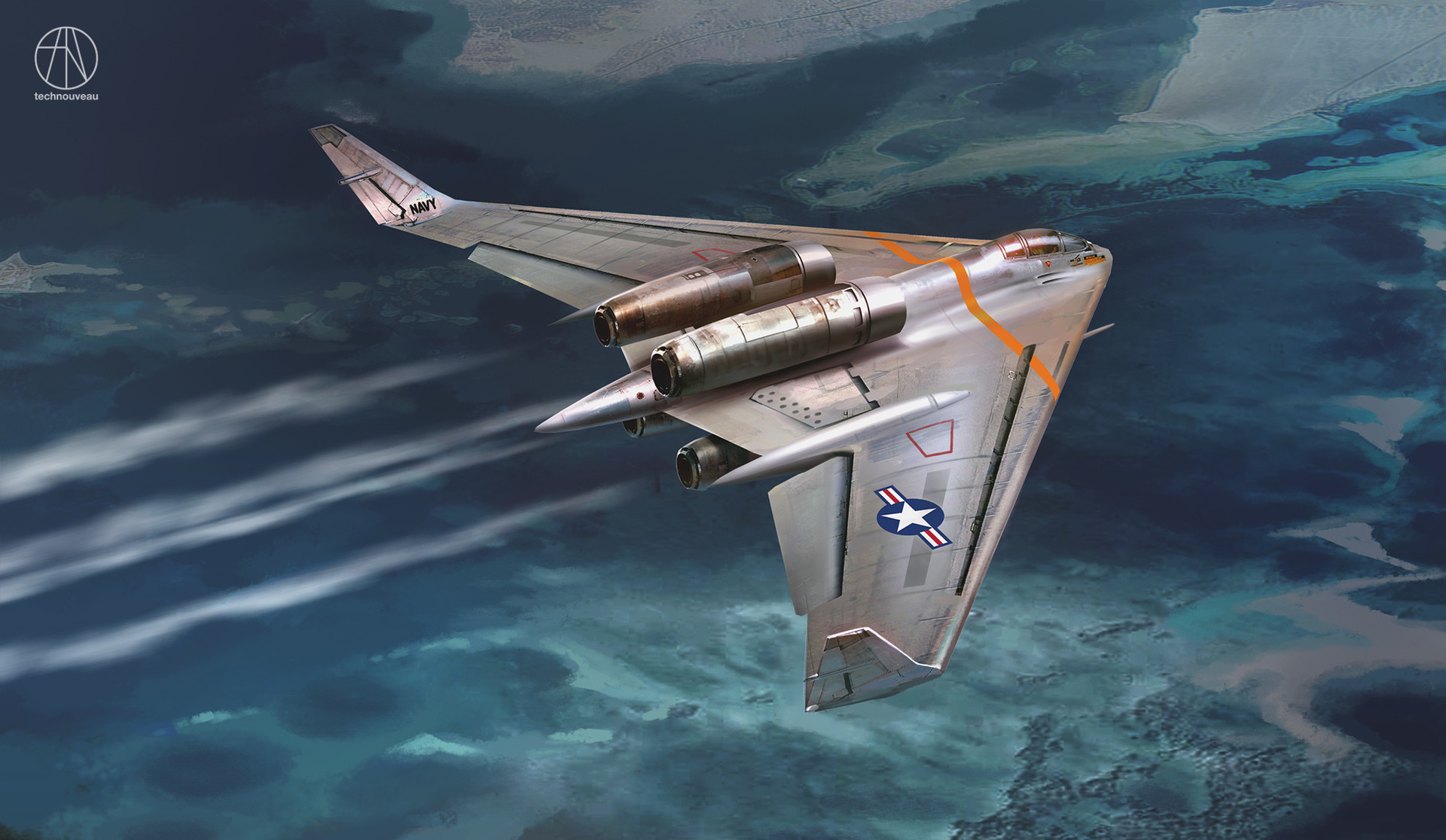A detailed digital render showcases a sleek, triangular stealth bomber, coated in a gleaming silver color. The aircraft, seemingly a 3D model or meticulously crafted concept art, features two prominent jet engines on its rear emitting vapor trails, and two additional smaller engines underneath. Its wings subtly curve upwards at the edges. Adorning the right wing is a distinctive emblem: a blue circle with a white star, flanked by red and white stripes, reminiscent of a Top Gun insignia, indicating its association with the United States. The plane is depicted flying over a scenic expanse of blue waters, flecked with white-capped mountain ranges or islands, hinting at diverse topography below. In the upper left corner of the image, a logo reads "Techno Nouveau," adding a futuristic touch to the visual narrative.